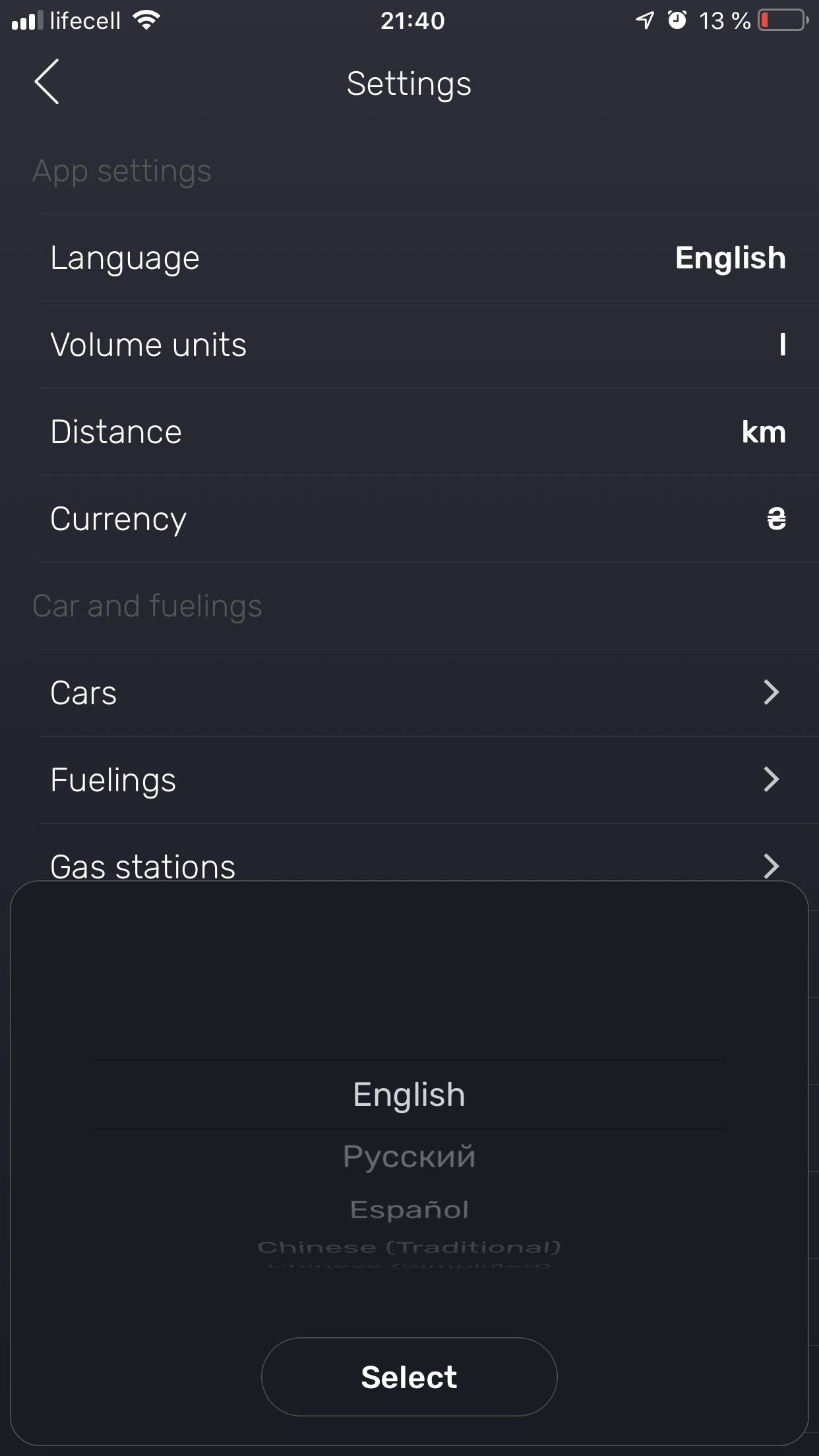This is a screenshot of the settings section within a mobile app designed for mile tracking. At the top, the header reads "Settings" in small, white letters. Beneath this header, various settings options are listed, including "Language," "Volume Units," "Distance," and "Currency." After a double spacing, the list continues with "Cars," "Fuelings," and "Gas Stations," each accompanied by an arrow on the right, indicating the availability of additional options or a dropdown menu.

In the bottom center of the screenshot, there is a scrolling selector for different languages. The first language listed is English, highlighted in white, denoting that it is currently selected. Angled slightly below are additional language options. At the very bottom of the screen, there is a bold, white button labeled "Select," allowing the user to confirm their language choice. The interface is designed to be intuitive, providing easy-to-access customization for various settings related to mileage tracking and vehicle management.